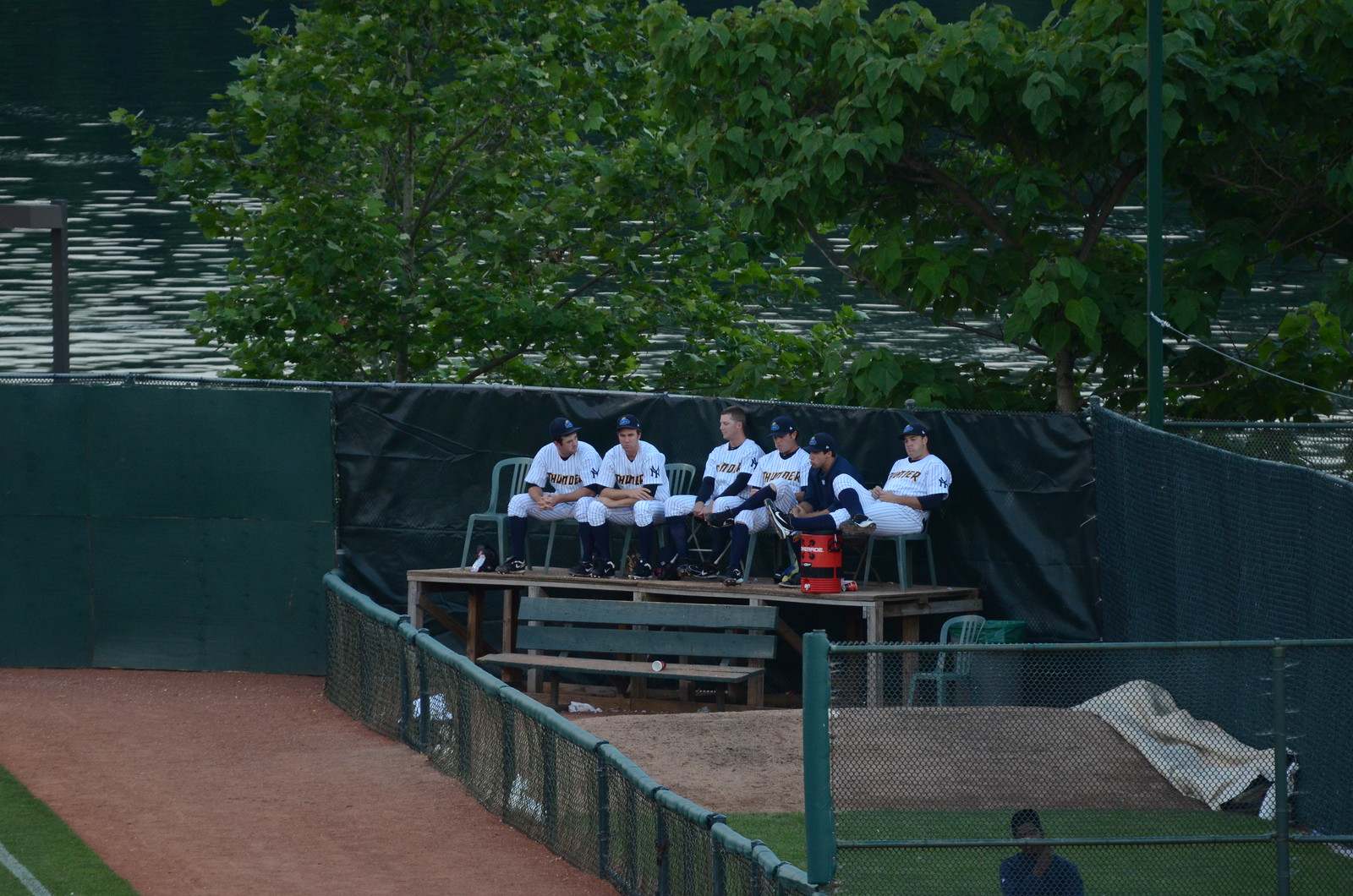The photograph captures a group of baseball players seated on green chairs arranged on a wooden platform, with a green bench below them. The players, wearing white, striped uniforms with "Thunder" written on the front and blue baseball caps—with the exception of one player—are situated in the corner of a fenced, enclosed area characteristic of a baseball field. Surrounding the players are a green wall and a green fabric-covered fence, with a strip of grass and dirt visible in front of the fence, indicating the boundary of the playing field. Behind the green enclosure, several trees can be seen, with a rippling body of water, likely a lake or river, further in the distance. The setting, marked by its rich green hues and the players positioned centrally, suggests an outdoor baseball park bathed in daylight.